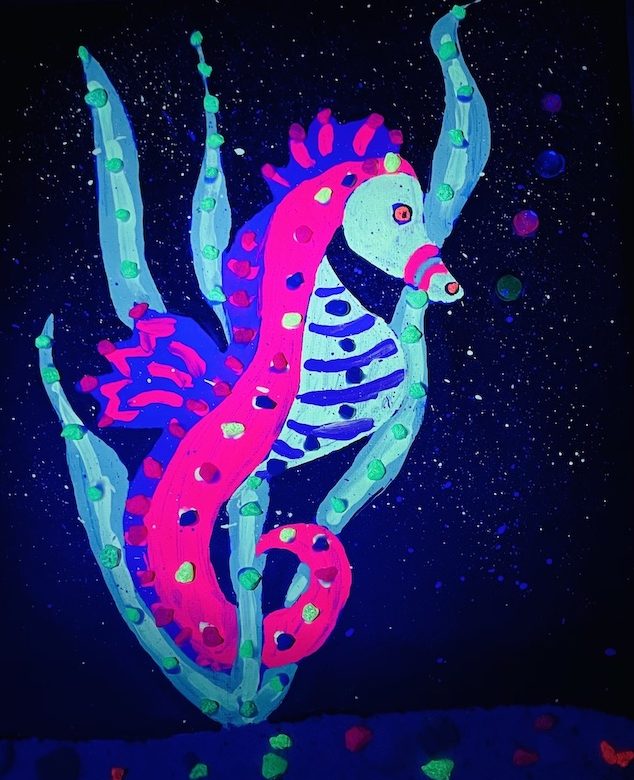This image appears to be a computer-generated artwork or painting, utilizing vibrant, black light-style colors to bring out its details. The focal point is a striking seahorse winding through pale teal seaweed or algae. The seahorse, shown in profile facing the right, boasts a dynamic color palette with neon pink, purple, and teal hues, complemented by a light blue belly adorned with horizontal blue stripes. Its face features a combination of blue and pink stripes around the muzzle, enhancing its fantastical appearance. Accenting its back are purple fins with pink stripes, and its midsection to the curled tail exhibits a gradient of pink, dotted with red, yellow, and black specks. Surrounding the seahorse is a dark, predominantly black background that mimics a starry night sky, speckled with white and featuring luminous colored bubbles in the upper right-hand corner. This striking contrast further accentuates the seahorse's glowing, surreal quality, making it appear almost illuminated by a black light.